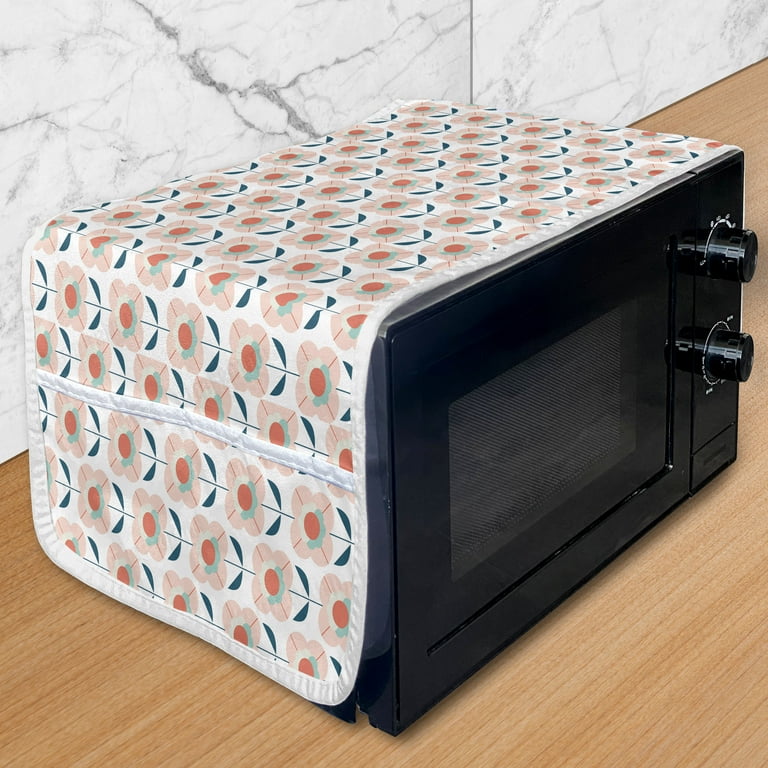The image depicts a small, vintage-style black appliance that could either be a microwave or toaster oven, featuring two manual turn dials instead of digital controls and a large push-button to open the door. The appliance sits on a tan wood grain countertop and is topped with a floral dust cover, which displays a pattern of pink, taupe, and two shades of green daisies against a white background, finished with white piping. The backdrop showcases a marble-like or terrazzo-style tile, suggesting a synthetic material. This diminutive heating device appears suitable for small dishes or single items and stands out against the detailed, polished kitchen setting.